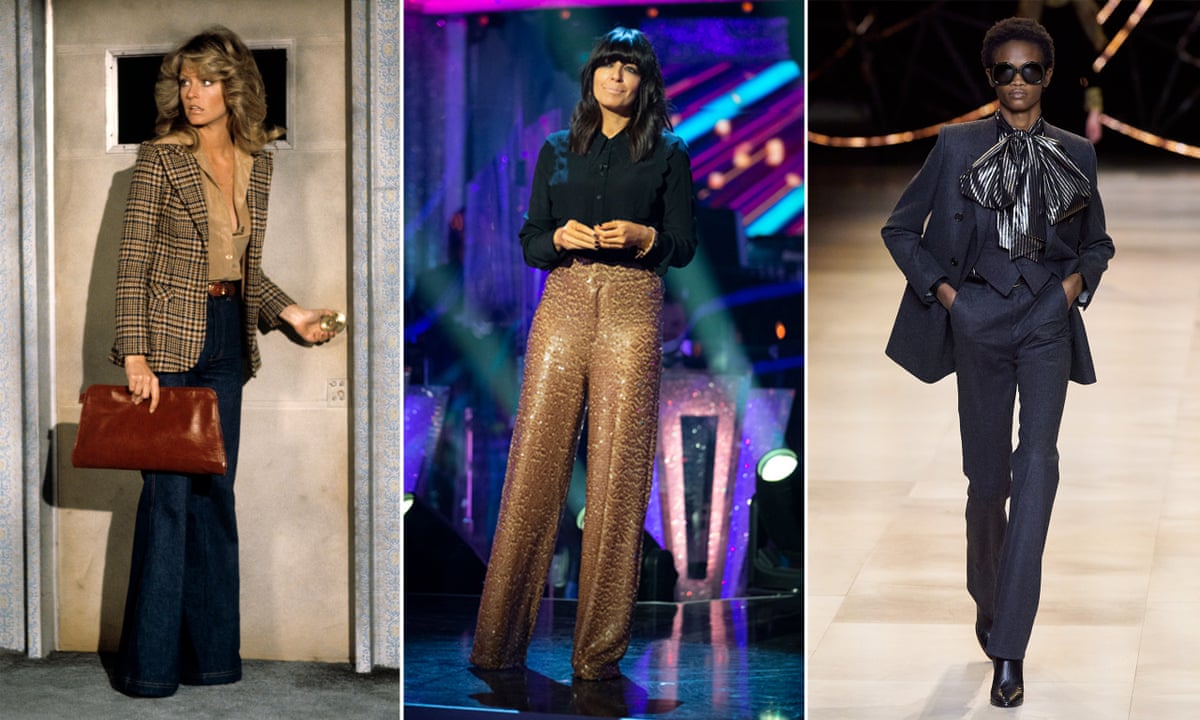The image showcases three distinct vintage photographs featuring women modeling outfits, each with a notably 1970s or early 1980s flair. On the left, Farrah Fawcett, recognizable from her Charlie's Angels days, sports a business-casual ensemble with an open vest over a brown shirt, wide-leg jeans cinched with a brown belt, and a red bag in hand as she opens a door. Her iconic, voluminous dirty blonde hair adds to the nostalgic feel. The woman in the center, likely a singer, flaunts black, glittery long-sleeve top paired with shiny golden speckled pants that are loose at the bottom, striking a pose that suggests she’s on stage. The final image on the right features another woman in a disco-retro look, complete with a flashy black suit adorned with a large black and white striped bow, accessorized with black sunglasses, and walking with a runway strut, her attire blending muted browns, blues, purples, and greens. Together, these photos create a vivid tableau of vintage fashion, characterized by bold styles and iconic materials.